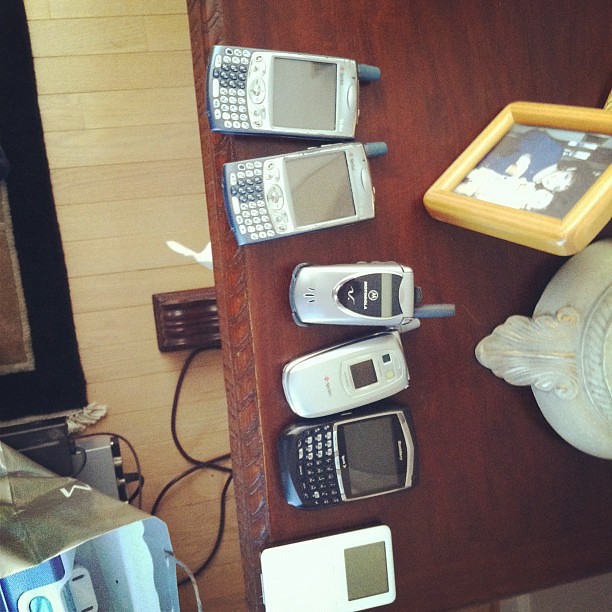This image captures a nostalgic scene imbued with retro and dated elements, primarily characterized by an assortment of old mobile devices such as two BlackBerries, a white iPod, two flip phones—one possibly a Motorola—and two silver PDAs with thick gray antennas and greenish-brown screens. These devices are meticulously lined up on a dark, reddish-brown wooden table that features intricate texture engravings on its sides. The table's vintage aesthetic is complemented by a grainy photo quality reminiscent of older cameras.

Adjacent to the electronics, a yellow picture frame holds a somewhat faded photograph of a woman with a child, evoking memories of the 80s or 90s. The table's surface also accommodates some pottery and a visible, open bag with undistinguishable contents. Below the table, electrical cords run into an outlet next to a blondish-colored wooden floor partially covered by a carpet, contributing to the overall retro ambiance. The image, captured from an overhead perspective, offers a snapshot of technological and personal history, merging the charm of yesteryears with the tactile presence of early mobile device technology.